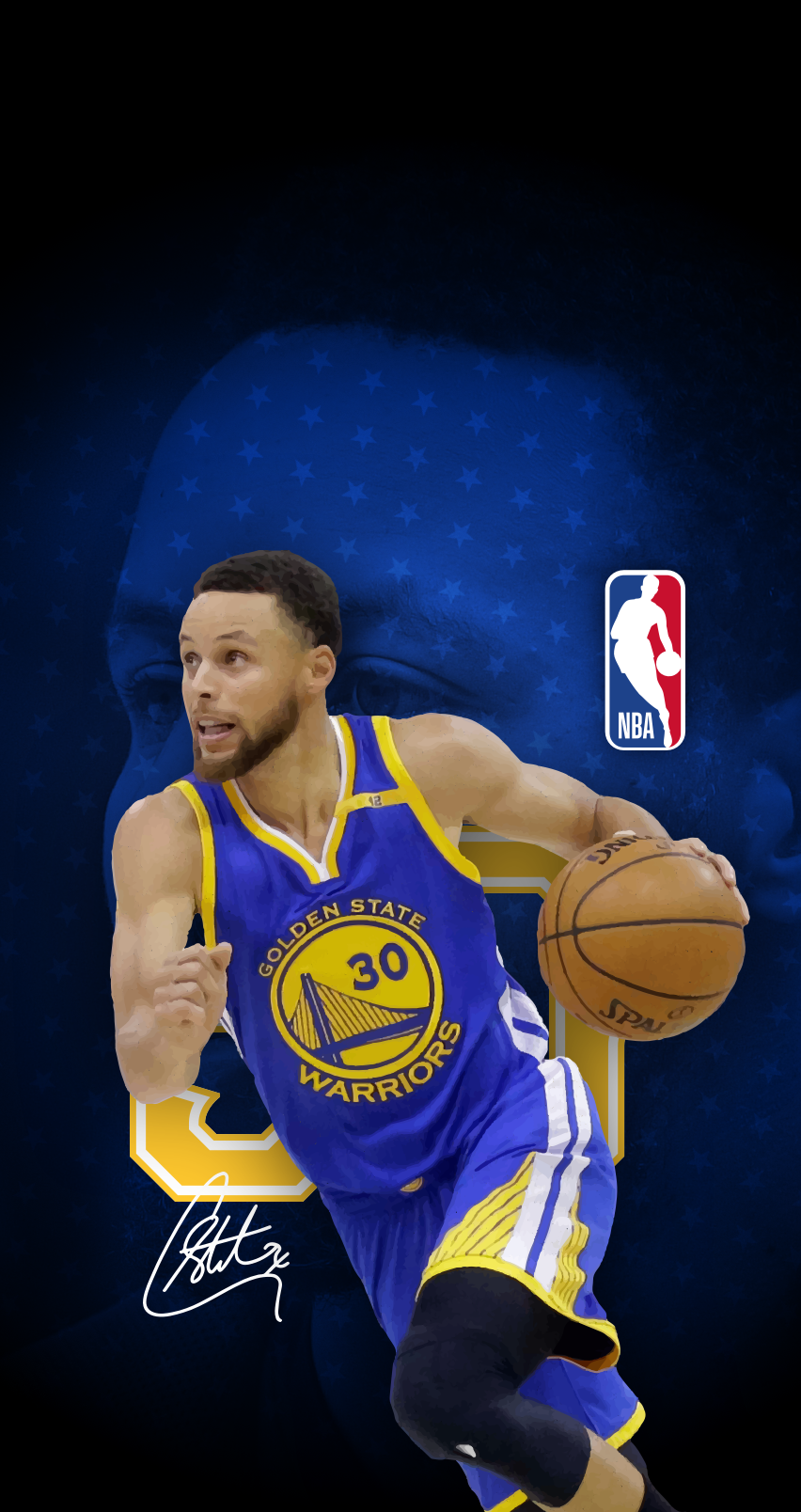This photograph captures NBA star Stephen Curry of the Golden State Warriors in action. Curry, wearing the iconic blue Golden State Warriors jersey with yellow trim and the number 30 emblem inside a gold circle featuring the Golden Gate Bridge, is seen dribbling a Spalding basketball with his left hand. His jersey, which commemorates the 30-year anniversary of the team's insignia, includes an NBA logo on the top right and Curry's distinctive white signature at the bottom left. The player sports black leggings under blue shorts adorned with white stripes featuring a blue central stripe. The image's background contrasts dark blue hues at the top and bottom with Curry's face centrally highlighted in a blue filter and adorned with lighter blue stars, creating a celestial effect.